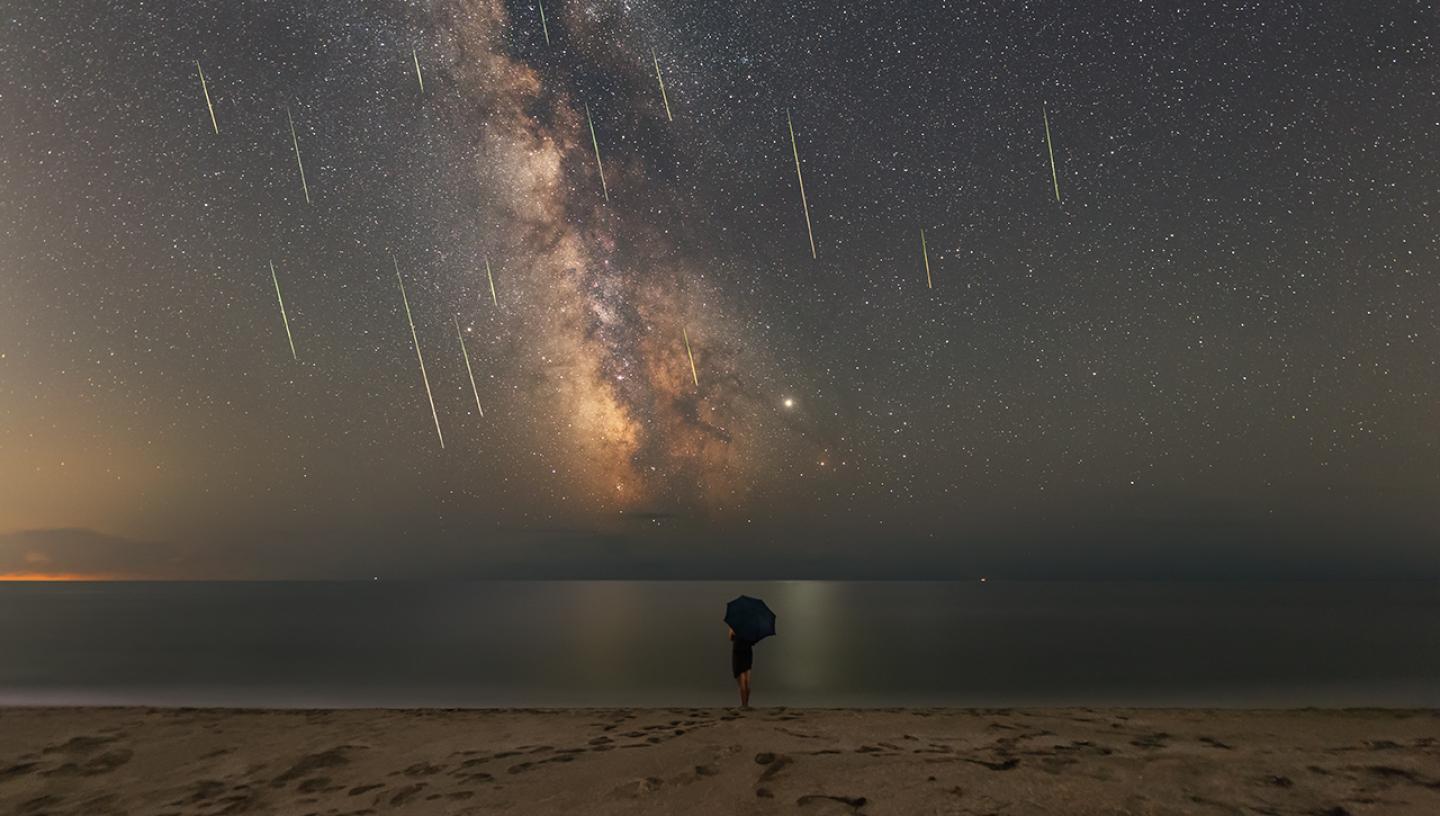In this stunning, high-quality nighttime photograph, the scene unfolds on a serene beach with dark brown sand that leads into a quietly lapping ocean, rendered in deep, metallic gray hues. Dominating the sky above is a breathtaking, galaxy-like vista, replete with countless white specks indicating distant stars, interspersed with streaks of falling or shooting stars that seem to cascade towards the horizon. Central to the image stands a solitary figure, merely a silhouette against the expansive night, dressed in black and holding a black umbrella, intently gazing out over the water towards the luminous stellar display. The captivating skyscape is lit up by an ethereal brightness, accentuating the Milky Way, making this image not only aesthetically pleasing but also profoundly evocative.